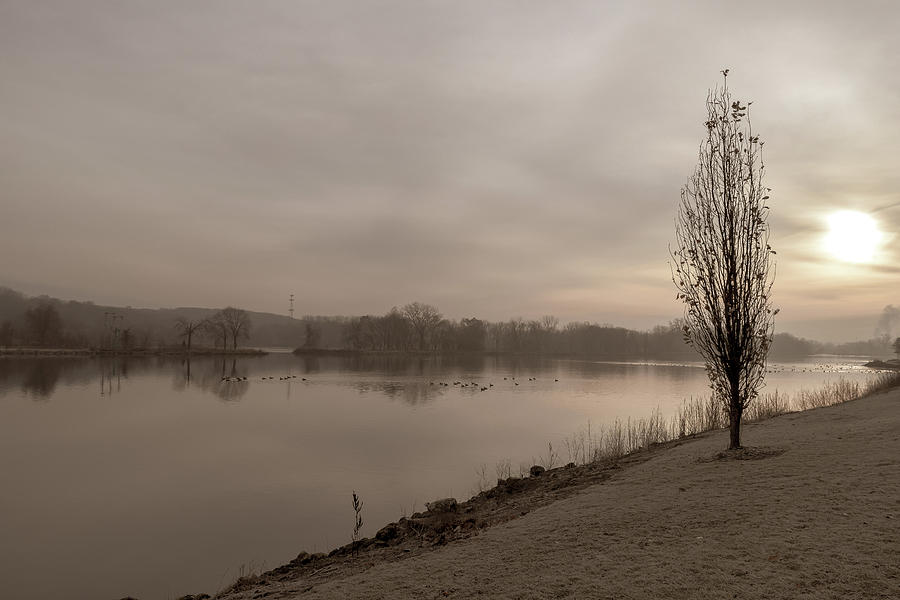The image captures a very wide river under a somber, overcast sky dominated by heavy gray clouds. The water, still as glass, reflects the dull ambiance. Along the riverbank, the grass appears brown and lifeless, typical of late autumn or winter. A tall, narrow tree with sparse leaves stands close to the river, its barren branches home to several small birds. Rocks scatter along the edge of the bank, enhancing the rugged feel. In the water, a few birds, likely ducks or geese, float peacefully. Across the river, an island with dead-looking trees can be seen, beyond which a mountain range extends from left to right, topped with a cell phone tower. The sun, a small white orb, sets near the horizon, casting subtle pinkish-gray hues across the sky and adding a faint peach tint to the overall scene. The right side of the image features a conical tree, and despite the dim lighting and depressed weather, the landscape evokes a tranquil, somber beauty.